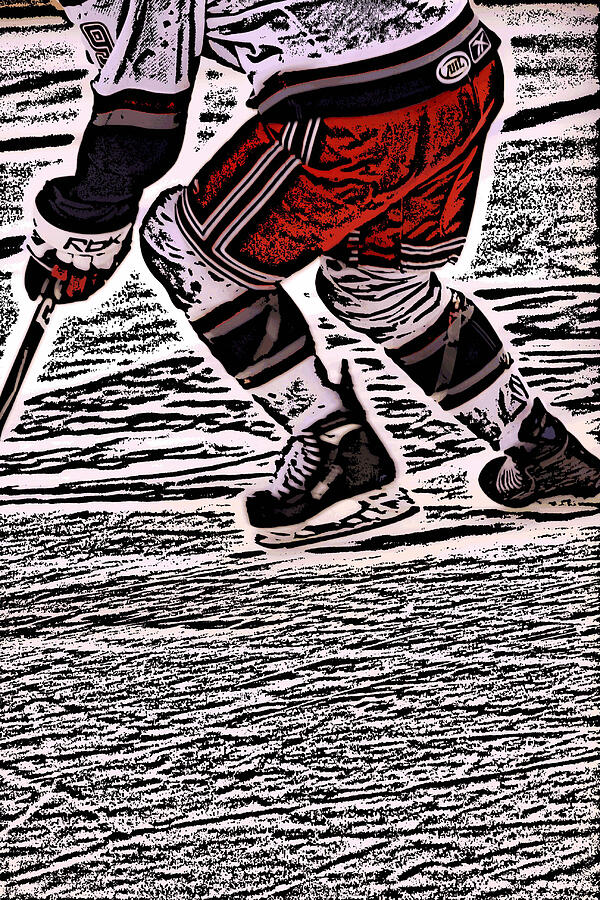The image is a stylized illustration of a hockey player skating on ice. The player is shown from the shoulders down, with no face visible, adding to the illustration-like effect. He's in motion, possibly hitting a puck, though it's not visible in the image. His equipment includes black skates with white laces, reddish-orange shorts with a black waistband featuring a gray strip, and black knee pads. The player wears a white jersey with the number 9 on the left shoulder. His gloves are branded with "RBK." The stick is black with a "G" on it. The scene is set against a predominantly white and black background, which is consistent with the filtered, artistic look of the image. There are some unreadable logos on the shorts and gloves. The skates are centrally placed in the composition, both vertically and horizontally, while the upper part of the body extends off the top edge of the frame. The ice surface beneath is white and black, hinting at a dynamic, possibly digitally altered, scene in an ice skating rink.